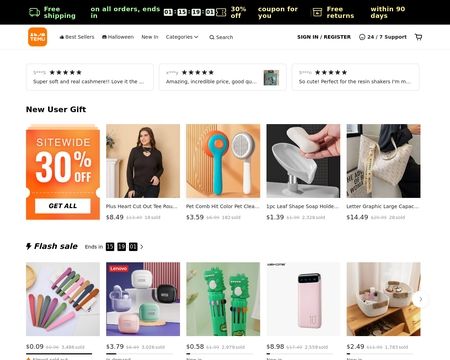This is a web page from TEMU. Across the top of the screen, there is a black ribbon featuring the text "Free shipping on all orders" in white. Adjacent to this, a countdown timer displayed within white boxes indicates "1 day, 15 hours, 19 minutes, and 1 second" remaining. It also mentions a "30% off coupon for you" and "Free returns within 90 days."

Beneath the ribbon, the background transitions to white. An orange square with the word "TEMU" in white is prominently placed on the left. The navigation bar runs across the top and includes the following categories: "Bestsellers," "Halloween," "New In," "Categories," "Search," and, on the far right, "Sign In/Register," "24/7 Support," and a shopping cart icon.

Further down, three horizontal rectangular boxes feature star ratings and customer text reviews. Below these, bold black text reads "User Gift," along with an orange box stating "Site-wide 30% off" in white text. Next to it, a white box invites users to "Get All."

The page continues with two rows of product images, each displaying prices and descriptions, offering a detailed visual assortment of the items available for purchase.